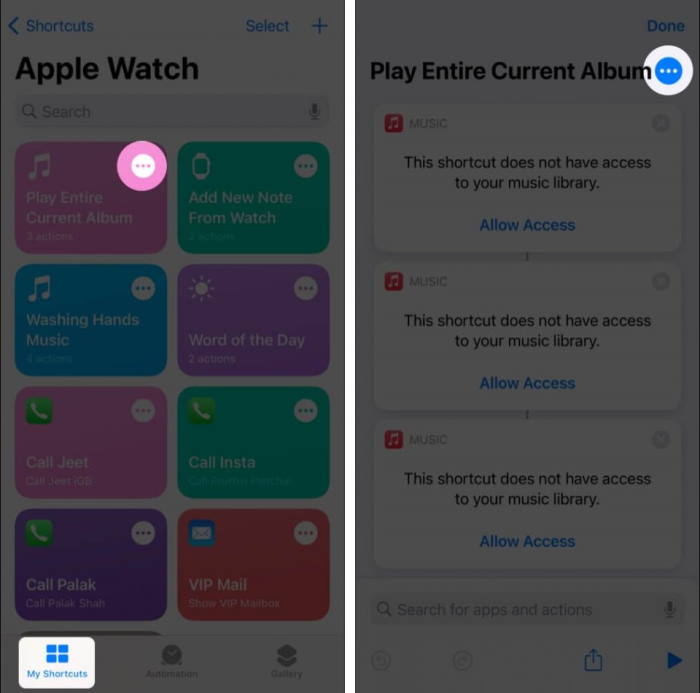This image is divided into two equal sections, left and right. The right section features a spotlight effect highlighting a circular area with three white dots in the top-right corner. 

The left section is more detailed and spotlights two areas: the same circle with three dots as seen in the right section, and the "My Shortcuts" button located at the bottom-left. Positioned centrally at the top of this left section, the text "Apple Watch" is displayed in black font. In the top-left corner, the word "Shortcuts" is accompanied by a left-pointing arrow, while the top-right corner features the word "Select" next to a plus sign.

Below the "Apple Watch" title, a search bar contains the word "Search" with a magnifying glass icon to its left and a microphone icon on the far right. The main body of this section consists of eight color-coded boxes arranged in four rows of two. 

From top to bottom, left to right:
- The first box is pink, labeled "Play Entire Current Album."
- The right box says "Add New Notes From Watch."
- The second row has "Washing Hands Music" on the left and "Word of the Day" on the right.
- The third row shows "Call Jeet" on the left and "Call Insta" on the right.
- The last row contains "Call Pellick" on the left and "VIP Mail" on the right.

At the bottom of this left section are the options "Automation" and "Gallery."